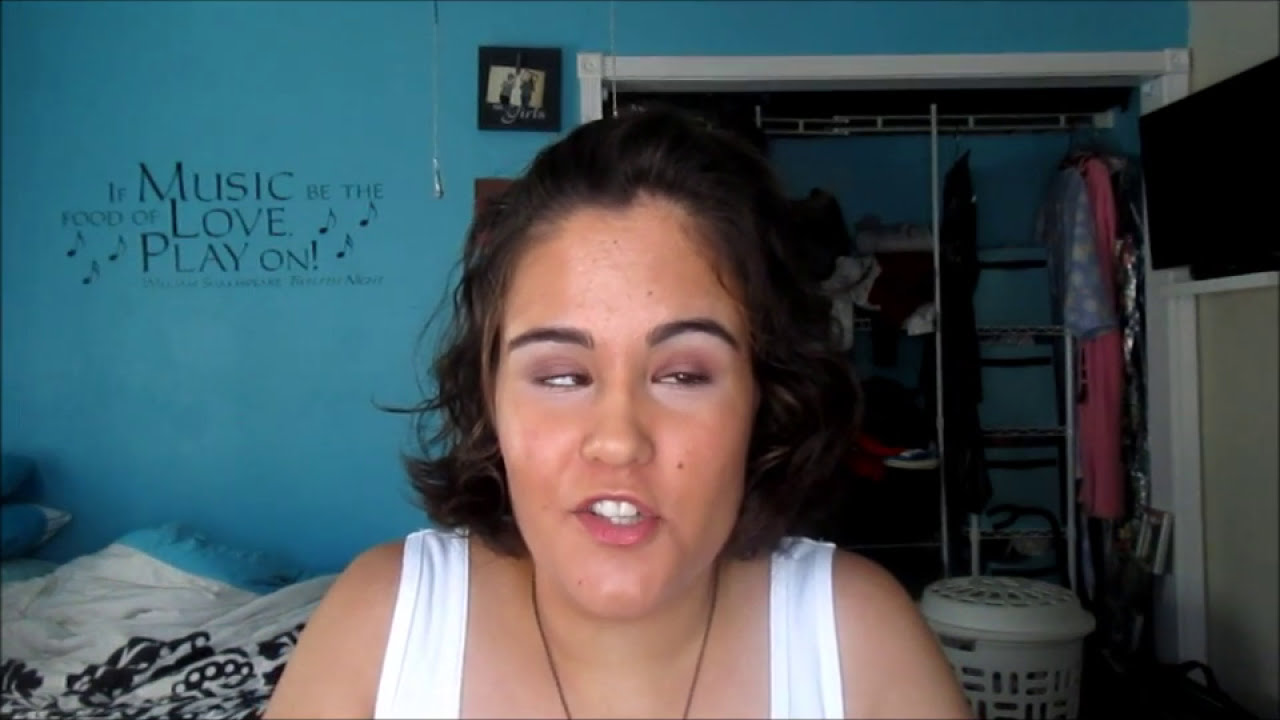The photograph captures a bedroom scene with two distinct colored walls: a blue back wall and a beige side wall. Dominating the right side is a TV propped up on a white shelf against the beige wall, which is turned off. Adjacent to the TV is an open closet filled with hanging clothes and some haphazardly tossed around; in front of this closet stands a white laundry hamper with a lid.

On the blue back wall, on the left side, a decal with the quote "If music be the food of love, play on" and musical notes decorates the space above a bed. The bed features a black and white bedspread with an additional white cover that has bluish edges.

Positioned in front of the closet and near the wall decal, a girl with short, curly brown hair tied back at the top is sitting and appears to be mid-sentence. She is wearing a white tank top that reveals her shoulders and part of her torso, and a black necklace is partially visible. Her eyes are half-closed as she looks to the left, her mouth slightly open with her teeth showing.